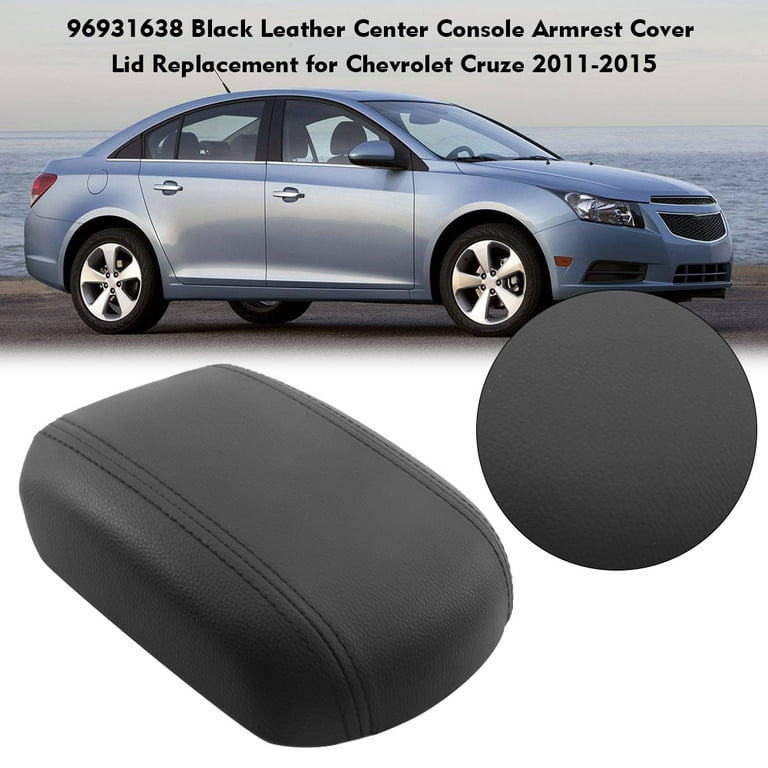This advertisement poster features a light blue Chevrolet Cruze, model years 2011 to 2015, shown in a side view parked on asphalt with a calm ocean in the background. At the top of the poster, in black text, it reads "969-31638 Black Leather Center Console Armrest Cover Lid Replacement for Chevrolet Cruze 2011-2015." Below this photograph, two detailed images of the replacement armrest cover and lid are overlaid. The armrest cover is cuboidal with curved edges, while the lid is circular, both made from fairly matte black leather with visible vertical stitching. The clean, new look of the car and its shiny hubcaps accentuate the high-quality, stylish replacement parts. The background of the entire poster is white, highlighting the text and images effectively.